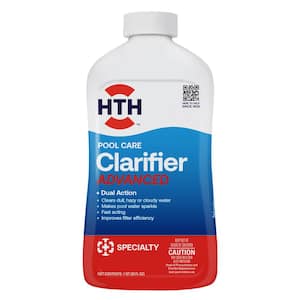This image depicts a plastic bottle of Clarifier Pool Care, designed for pool maintenance. The bottle's top part, including the white cap, displays a QR code on the upper right side and a red, double-arched HTH logo with black lettering on the upper left. Below this white section is a blue middle portion, which features white text stating "Pool Care," with "Clarifier" in larger letters and the word "Advanced" in red text beneath it. This blue section also contains four or five white bullet points, detailing its benefits, though they are too small and blurry to read clearly. The bottom portion of the bottle is red, featuring a small white specialty symbol and the word "Specialty" next to it, with some fine print on the right side, including a readable "Caution" notice. The overall backdrop of the image is plain white, emphasizing the bottle’s distinctive tricolor design of white, blue, and red sections.